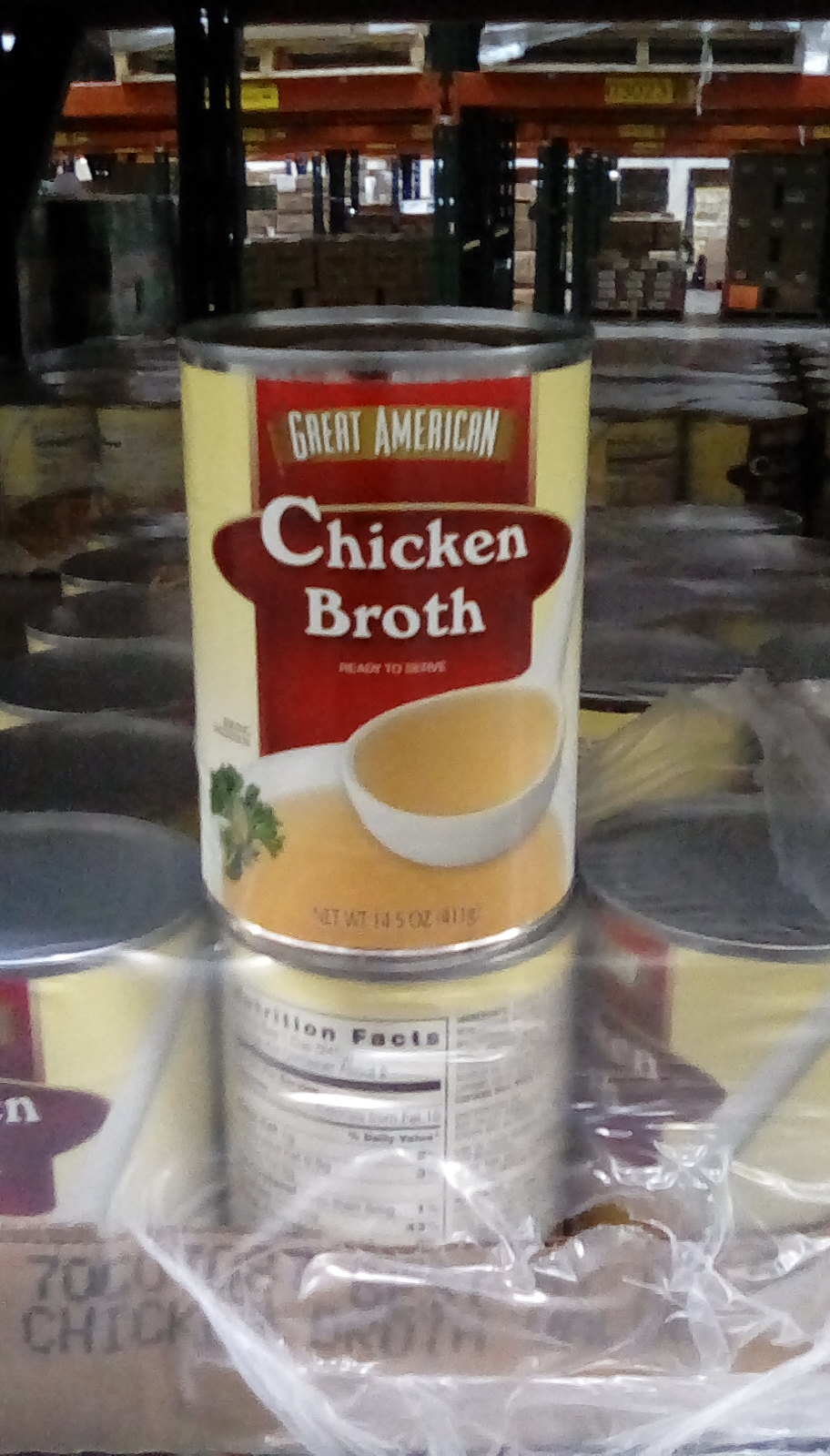This is an image of a can of Great American Chicken Broth displayed in a warehouse setting. The can features a light beige and red label, with the brand name "Great American" prominently displayed at the top, followed by "Chicken Broth" in white letters within a dark red rectangle. Below the text, the label depicts a white bowl filled with tan-colored chicken broth, accompanied by a white ladle dipped into the soup, and a small garnishment of green herbs to the left of the bowl. The can itself is aluminum with a shiny gray top. It is positioned atop a case of identical cans, which are packaged in plastic wrap, and the surrounding environment suggests a storage area within a warehouse, ready for shipment to retail stores.